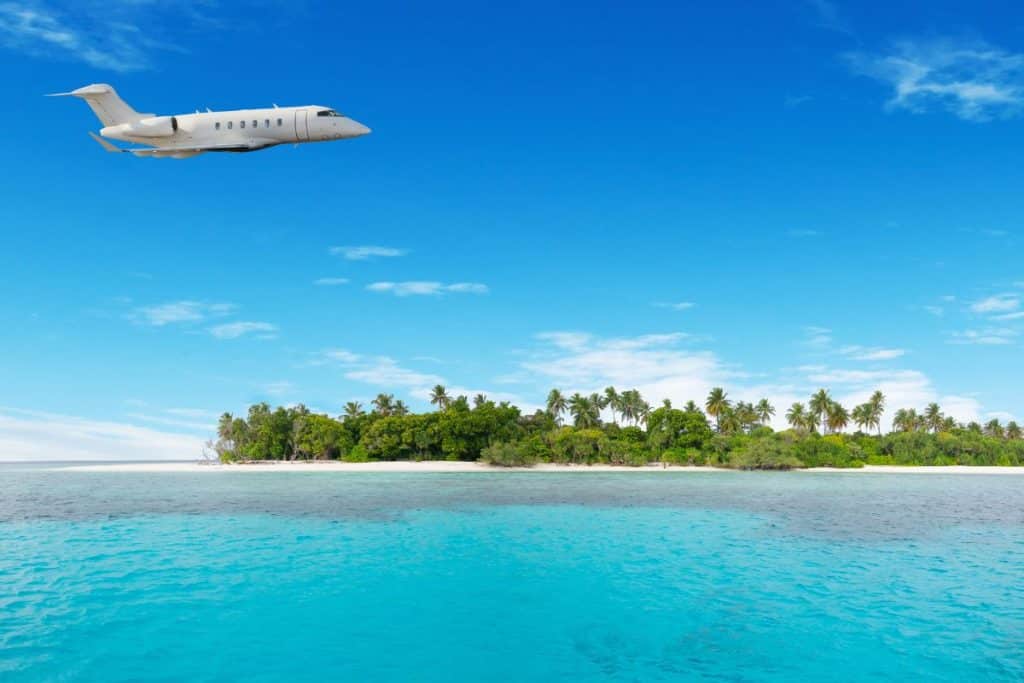This captivating daytime photograph showcases a vibrant tropical scene. Dominating the left side of the picture, a sleek, white business jet with six windows and two engines can be seen soaring across a gradation of cyan to dark blue ocean waters. The jet, featuring a bay door for disembarking, flies from the left towards the right, poised against a backdrop of a cyan-blue sky decorated with splotches of white, wispy clouds.

Beneath the jet, the serene waterway starts with a bright aqua hue, progressively deepening to a rich navy blue as it approaches a small island. This island, characterized by its pristine white sandy beaches, is richly adorned with lush greenery. Tall trees, including palms and possibly evergreens, rise prominently, accompanied by large green bushes that line the landmass, which extends out of the picture frame on the right. The juxtaposition of the cyan sky, multicolored ocean, and verdant island creates a stunning visual narrative of an untouched, picturesque tropical paradise.